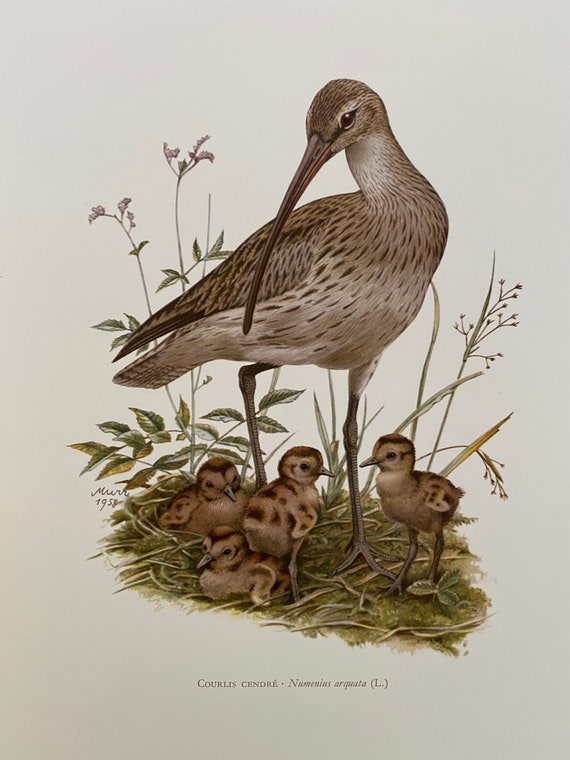This is a detailed illustration of a bird, identified as Coralis cendrei (Numenius arquata L.), with four chicks around its feet. The bird, which resembles a waterfowl and shares similarities with a hummingbird due to its long, slightly curved beak, stands prominently in the grass. Its overall coloration is a mix of beige or light brown with distinctive brown spots dispersed across its body and feathers. The wings and tail feathers are slightly darker, with a pattern of brown clusters toward the ends. The head of the bird is brown, transitioning to a more beige hue around the face. The chicks below, depicted in darker brown with stripes on their backs and brown-spotted wings, have short beaks. Behind the family, plants and flowers emerge from the grassy setting. This painting, created by Murr in 1958, captures the bird in a leftward gaze, focusing down at its chicks, while the body is oriented to the right.